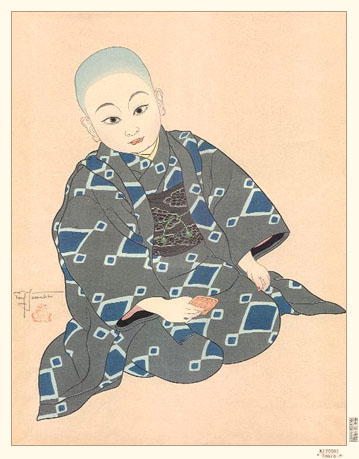The image depicts an oriental-style drawing or painting set against a solid light peach or salmon-colored background. The central figure is an androgynous young child kneeling, with very short hair and sporting a contemplative expression, neither happy nor sad. They have curved round eyebrows, almond-shaped eyes, small ears, and red lips. The child is clothed in a gray robe adorned with a pattern of blue triangles in varying sizes, resembling a kimono. Around their waist, there is a brown obi-like sash. The child’s right hand is holding what appears to be a cracker or a card, while the left hand rests relaxed at their side. The background features some illegible writing and a character on the left-hand side, adding to the oriental aesthetic of the scene. The figure directly engages the viewer with their gaze, adding a sense of intimacy and stillness to the composition.